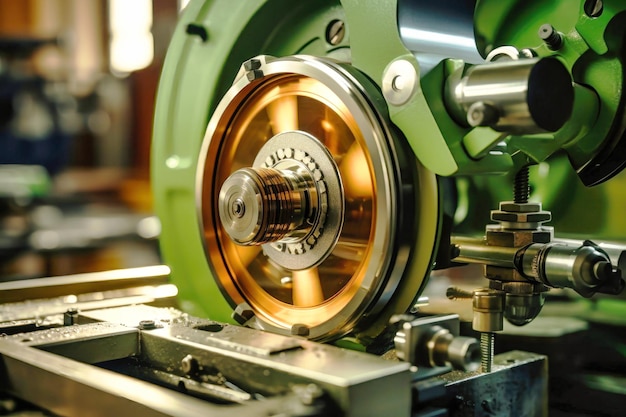This detailed photograph features a close-up view of a piece of machinery, likely in a workshop environment. Central to the image is a shiny, golden or copper-colored disc with a silver cylinder protruding from its middle, encased by a circular silver metal rim. This disc is part of a larger green metal machine. The green machinery includes various components, such as metal bars on the left which could be used to position materials for cutting, and possible drills on the right. The machine is mounted on a metal surface or frame with a silvery hue. The background of the image is intentionally blurred, rendering other workshop equipment and details indistinguishable, contributing to the overall focus on the primary tool. The image has a somewhat unrealistic, possibly AI-generated appearance, but maintains a realistic style overall. The golden disc and the green casing create a striking color contrast in an otherwise metallic silver and green palette. Despite the detailed depiction, the exact purpose of this tool remains unclear, though it hints at potential use in metalworking or possibly woodworking.